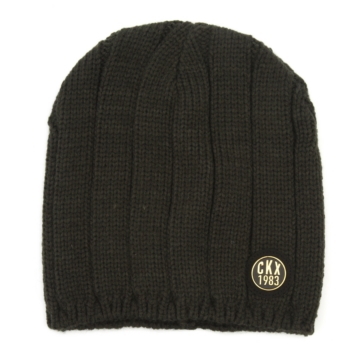The image depicts a dark green knit cap, commonly referred to as a beanie or toboggan hat, lying flat on a white background. The cap features vertical, one-inch parallel lines running from the top to the bottom, providing a distinct pattern. At the bottom, there is an elastic band to secure it on the wearer’s head. In the lower right-hand corner of the hat, there is a small circular logo button with the inscription "CKX 1983" outlined in white, suggesting either the brand name or the year of establishment. This detailed product photograph appears to be intended for a website or catalog.